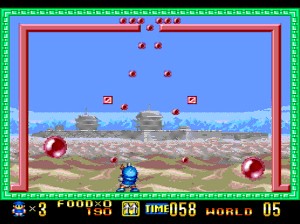This image is a screenshot from a video game. The interface features a green rectangular border framing the main play area. Below this green boundary, the bottom section of the screen is set against a black background. Moving from left to right in this bottom area, there's a small logo depicting a character dressed in blue clothing, followed by an indicator showing "x3," which likely denotes the number of lives or character count. Next, there's a "food x0" indicator, implying the current amount of food collected. The numbers "190" possibly represent the player's score or points accrued. Time display reads "058," potentially indicating the time left or elapsed in the game. The label "world 05" suggests the current level or stage within the game. In the main gameplay area, a cartoon character stands at the center, facing an oncoming barrage of red orbs descending from the top of the screen, likely representing obstacles or enemies the player must evade or overcome.